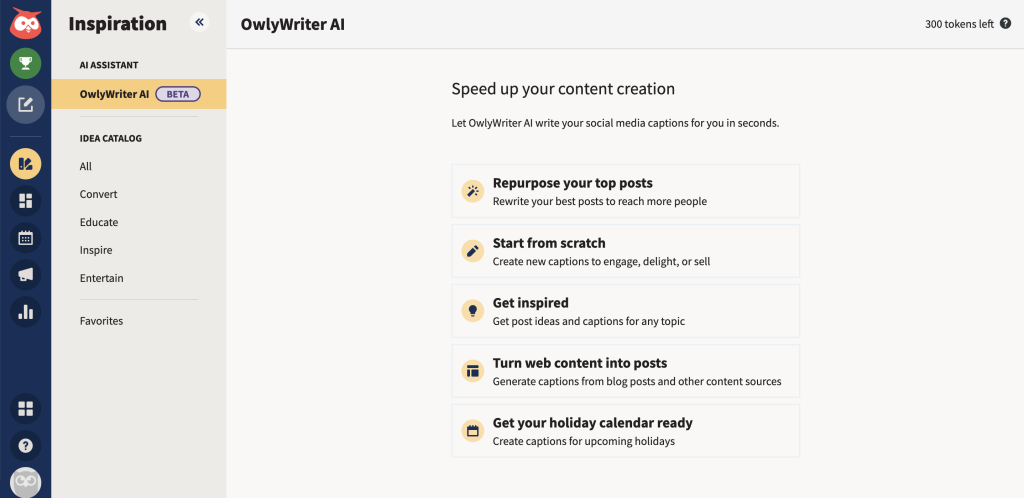### Descriptive Caption:

The image is a screenshot of a user interface with a light beige background. On the left, there is a navy vertical sidebar featuring several icons. From top to bottom, the icons include an orange owl, a solid green circle with a cup, a solid yellow circle (likely indicating the search function), and various other symbols.

Upon selecting a desired area to explore, a menu appears, displaying options such as "Inspiration," "AI Assistance," "Owly Writer AI Beta," "Idea Catalog," "All," "Convert," "Education," "Inspire," "Entertain," and "Favorites." Additionally, there are buttons to "Speed up your content creation," letting users allow Owly Writer to compose social media captions in seconds. Users are informed that they have 300 tokens left. Other options include "Repurpose," "Start from scratch," "Get inspired," "Turn content into posts," and "Get your holiday."

Adjacent to these textual prompts are solid yellow circle icons with black objects representing various functionalities. At the top of the interface, a question mark icon is visible alongside a promotional message: "Get your holiday calendar ready." This feature suggests creating captions for upcoming holidays, further emphasizing the search functionality described earlier.

This detailed layout effectively showcases the features and options available within the user interface.